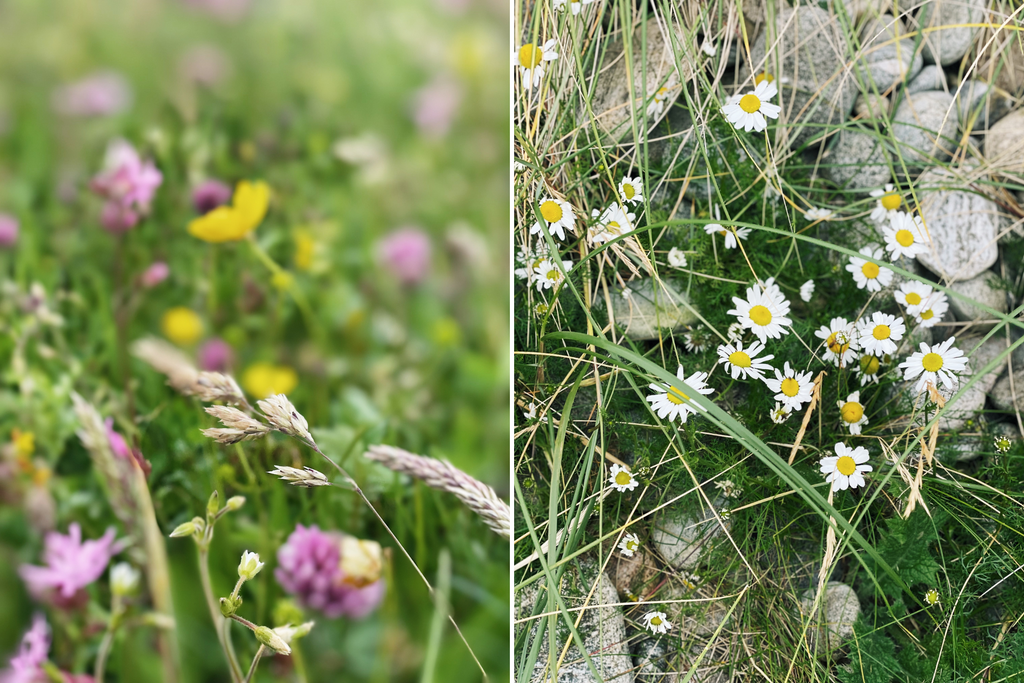This image is a side-by-side composition of two detailed, contrasting scenes of flowers in natural settings. On the left, there is a prairie or meadow with a mix of pink and yellow flowers, possibly accompanied by free-growing wheat or tares, all intertwined with vibrant green foliage. The background is deliberately out of focus, accentuating the natural environment with a touch of green amid the blurred flowers. On the right, a sharper image captures white flowers with yellow centers growing amidst green moss and gray rocks, likely along a rocky river shoreline. This half includes clear details such as scattered rocks and patches of yellow and green grass. Overall, the contrast between the blurred left side and the sharp right side creates a dynamic and picturesque dual representation of floral beauty in different natural habitats.